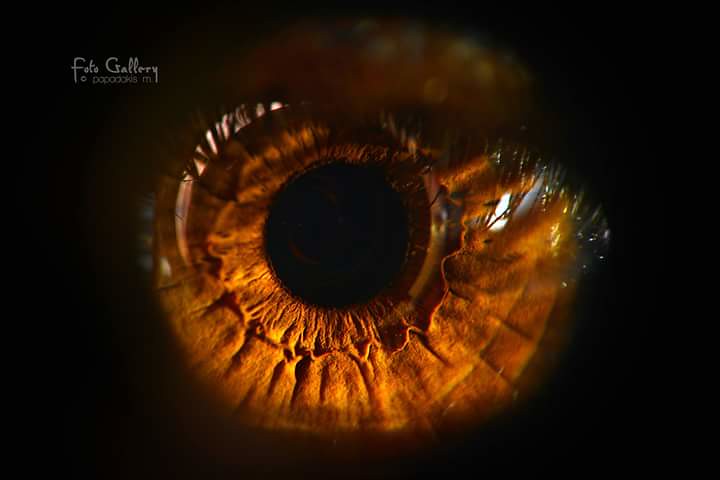This detailed macro photograph showcases the mesmerizing close-up of an eye's iris and pupil. Dominated by rich, amber, and golden hues, the intricately patterned iris features a jagged ridge forming a striking ring around the centrally placed, pitch-black pupil. The reflective quality of the eye's lens captures subtle reflections, possibly including the silhouette of eyelashes, against a stark black background. Above this captivating image, the text "Fate Gallery" appears in gray, adding an artistic touch to the striking visual. Each detail—from the shimmering golden tones to the illusion of depth within the eye—contributes to an almost otherworldly, yet intimately human, representation.